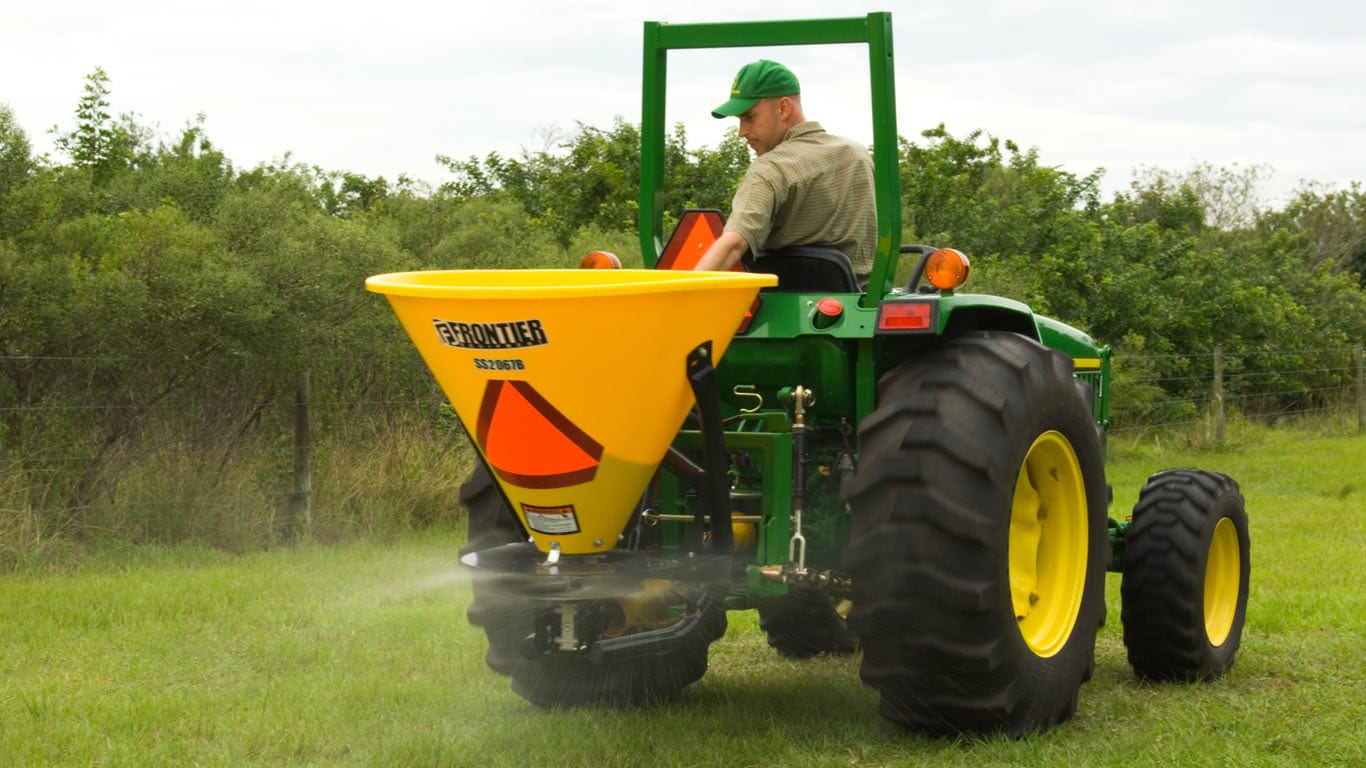In the photograph, a man is operating a small green John Deere tractor adorned with large black and yellow wheels. The tractor is equipped with several safety features, including a roll bar and triangular-shaped reflectors. The man, who is wearing a green John Deere hat and a tan short-sleeved shirt, is seated facing backward, concentrating on a yellow funnel-shaped hopper mounted on the tractor's rear. This hopper, labeled "Frontier SS 29678," is dispensing seeds or fertilizer across a lush, green lawn through a whirling mechanism. The scene is set against a backdrop of greenery and tall bushes under a cloudy sky. The active spreading of material creates a noticeable sense of motion in the image.